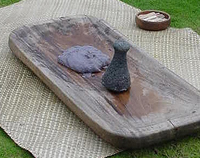In the image, we see a large tarp, beige in color, spread out on a backdrop of green grass, partially visible in the corners. Centered on the tarp is an older-fashioned, rectangular wooden plate, characterized by a worn, light brown outer edge and a more polished, stained middle. Atop the plate rests a bell-shaped, charcoal-black grinder, likely a heavy-bottomed pestle, indicative of an antique meal apparatus used for mashing food like corn. Next to it lies a flat, gray stone, possibly used in conjunction with the pestle. In the top right corner of the tarp sits a small, brown ring-shaped bowl containing several white objects, adding a subtle contrast to the scene.